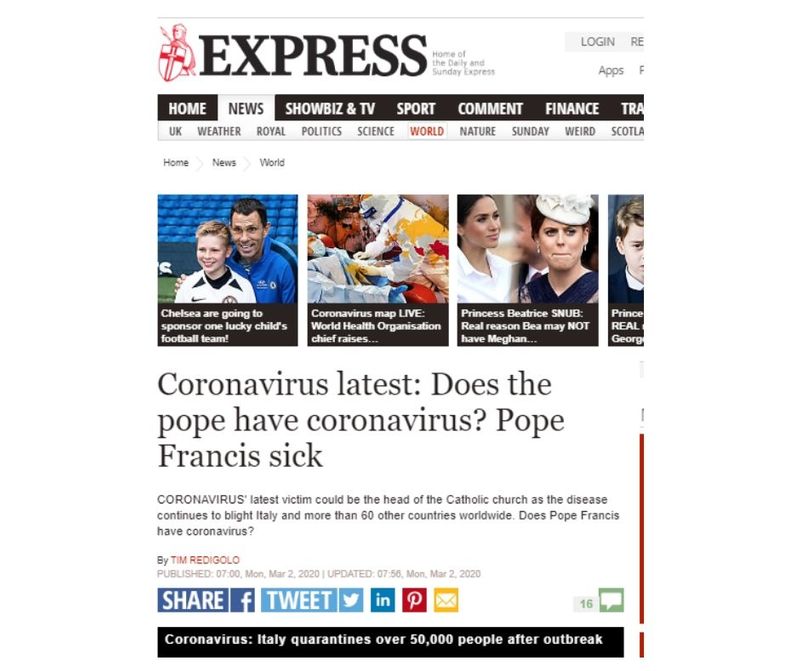This screenshot captures the homepage of a newspaper website with a clean white background, colorful thumbnails, and vibrant social media link icons. In the top left corner, there is a distinctive knight emblem holding a shield adorned with a red cross, positioned next to the bold, capitalized word "EXPRESS." 

On the top right, options to log in are clearly visible. Below this, the header bar prominently displays various sections: Home, News, Showbiz & TV, Sport, Comment, Finance, and Travel. The News tab is currently selected, highlighted in white, with subcategories listed just underneath. Among them are UK Weather, Royal, Politics, Science, World, Nature, Sunday, Weird, and Scotland, with the World tab highlighted in red, indicating your current selection.

A breadcrumb trail shows your navigation from Home to News to World. Below this, four notable thumbnails span the width of the top section:

1. An image of a boy with an adult football player, accompanied by text stating, "Chelsea to sponsor one lucky child's football team."
2. An image suggesting a hospital scene with the headline, "Coronavirus map live: World Health Organization chief raises..."
3. A photo featuring Meghan Markle and Princess Beatrice, with a headline hinting at, "Princess Beatrice snub - Real reason Beatrice may not have Meghan..."
4. A partial glimpse of Prince George.

Dominating the page is the main headline: "Coronavirus Latest: Does the Pope have coronavirus? Pope Francis sick." A subheading beneath provides additional context, noting the article's date, March 2, 2020. Social media sharing options including Facebook, Twitter, Pinterest, Email, and Comment buttons follow directly after the subheading.

At the bottom of the page, a bold black banner runs across, delivering urgent news: "Coronavirus: Italy quarantines over 50,000 people after outbreak."